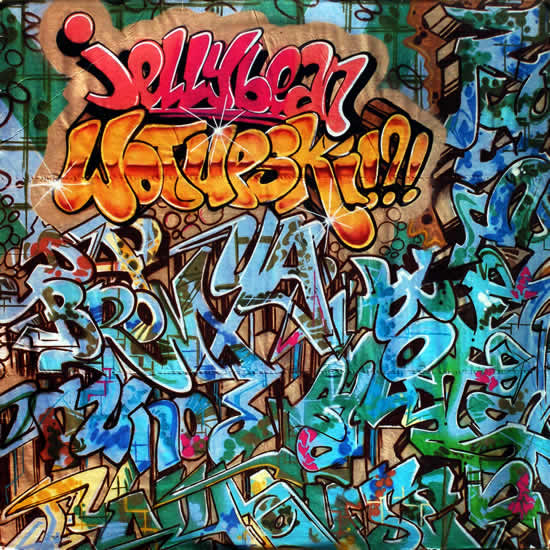This image showcases an intricate and colorful piece of graffiti art that occupies an entire wall. The mural features a vibrant mix of colors including predominant shades of blue, green, and brown, with additional accents of pink, orange, light blue, beige, and yellow. The central elements of the graffiti are words, some of which are clearly distinguishable while others are more abstract or obscured. Notably, the word "Bronx" and the letters "YA" can be seen amidst the chaotic background.

At the top left corner of the mural, the phrase "Jelly Bean Wotupski" stands out prominently. The words "Jelly Bean" are rendered in a striking red or pink color, while "Wotupski" is depicted in orange or gold. This phrase is punctuated with an exclamation point, a question mark, and another exclamation point, adding a dynamic flair. The overall image is vividly clear and well-lit, accentuating the graffiti's bright and varied color palette against a backdrop that transitions from light to dark hues. The entire scene is a testament to the energetic and eclectic nature of graffiti art.